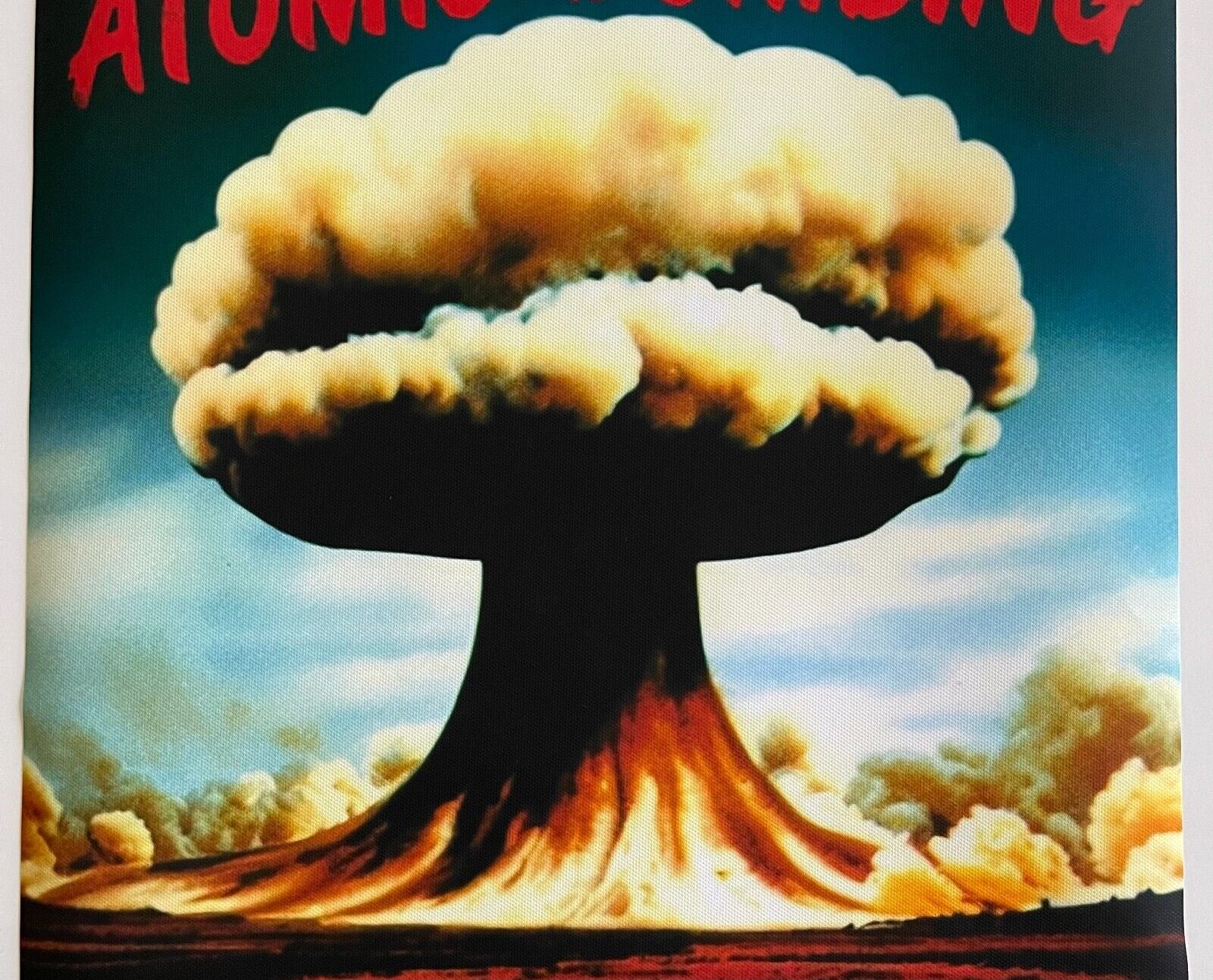This image appears to be of a poster, likely related to atomic testing. The top of the poster is partially cut off, but you can discern the red letter "A" on the top left, hinting that the word "atomic" is spelled out partially. A thin gray border frames the right and left sides of the poster. The central focus of the image is a large, brown mushroom cloud, typical of an atomic bomb explosion, rising prominently from the ground. The bottom part of the mushroom cloud is darker, almost black, while the middle and upper parts transition to yellow and brown tones. Surrounding the mushroom cloud, the sky has a mix of blue and white, with some distant white clouds visible. The ground beneath the explosion is dark and scorched. The entire scene is dominated by the mushroom cloud, which occupies most of the sky space, creating a stark contrast against the more tranquil clouds in the background.